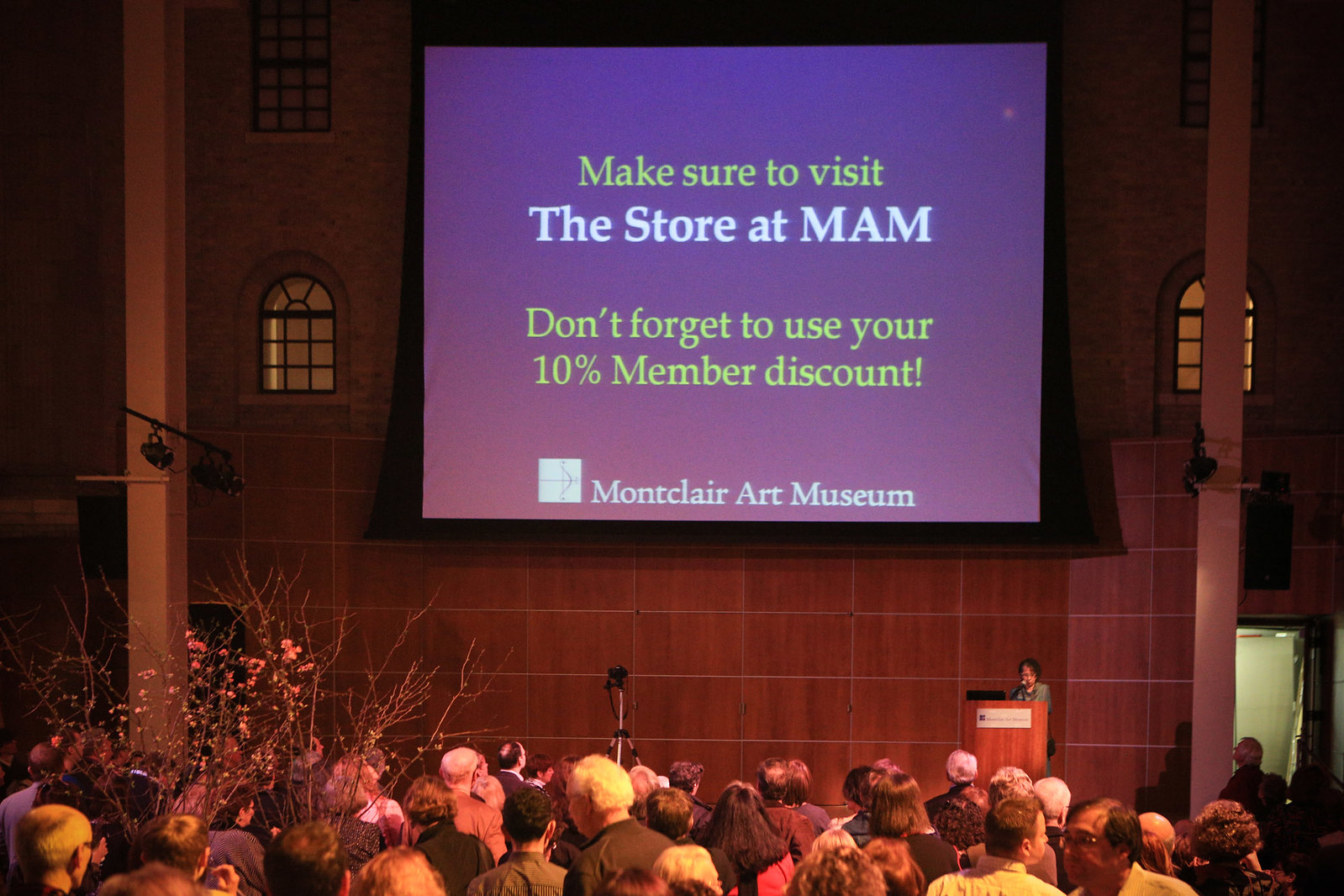In this color photograph, a large crowd of people, visible by their heads and shoulders, fills the lower portion of the image. At the center, there is a microphone placed in front of a podium, where a woman stands behind it, addressing the crowd. The scene is set indoors with a prominent stone wall in the background. Dominating the upper middle section of the image is a large projector screen with a blue background featuring a message in various colors. The text on the screen reads: "Make sure to visit the store at MAM. Don't forget to use your 10% member discount. Montclair Art Museum." Additional details include a window to the left of the screen and another to the right, each with a lantern hanging above, likely providing light. Further to the right of the podium, near the edge of the photograph, is a doorway with an open light on, adding to the scene's ambiance. To the left, a tree adorned with white flowers is partially visible, adding a touch of nature to the setting. Two columns on either side frame the photograph, encapsulating the event taking place.